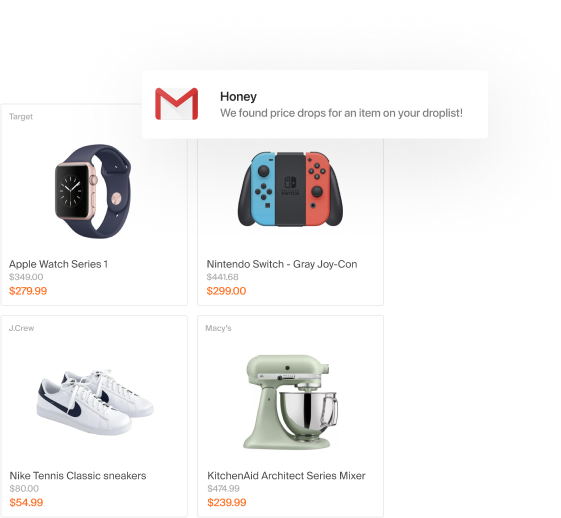This image features a screenshot displaying various product advertisements, showcasing discounted prices from different retailers. In the upper left corner, there are four product photographs with details:

1. **Apple Watch Series 1 from Target**: Originally priced at $349, now reduced to $279.99.
2. **Nintendo Switch Gray Joy-Con**: Initially priced at $441.68 and now available for $299.
3. **Nike Tennis Classic Sneakers from J.Crew**: Originally $80, now on sale for $54.99.
4. **KitchenAid Architect Series Mixer from Macy's**: Previously priced at $474.99, reduced to $239.99.

Additionally, there is a pop-up notification in the upper right corner from Honey, indicating, "We found price drops for an item on your drop list," accompanied by a mail icon on the left.